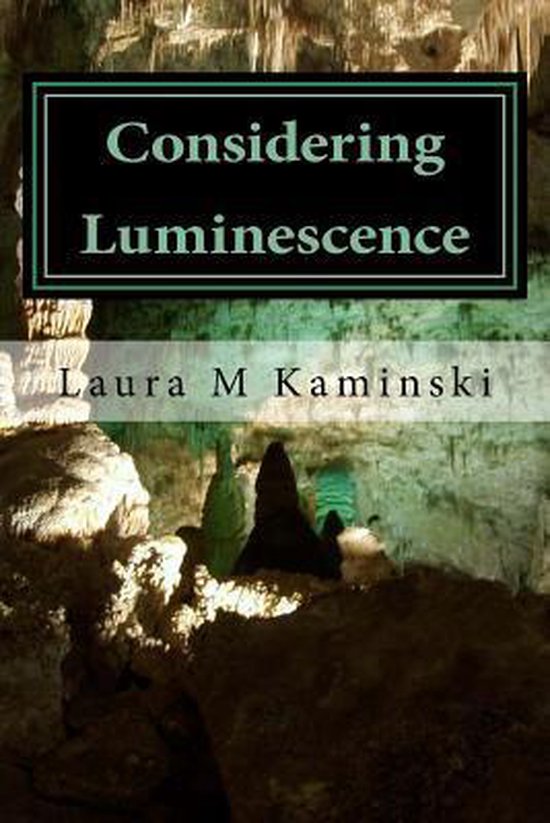The image is a photograph of a book cover. The top of the cover features the title "Considering Luminescence" written in a very pale green serif font, set inside a black box. This box has two borders: a dual-layered design with an inner light green border and an outer white border. Below the title, the author’s name, "Laura M. Kaminsky," is displayed in a Times New Roman-like black font on a semi-transparent white band. The background of the cover is an illuminated photograph of the inside of a cave, showcasing the natural formations of stalactites at the top and stalagmites at the bottom. The cave scene has brown accents with hints of green, possibly intended to complement the light green border of the title box, creating a visually cohesive design. The cave appears brighter towards the top and middle, with darker tones at the bottom, highlighting the interplay between light and shadows.